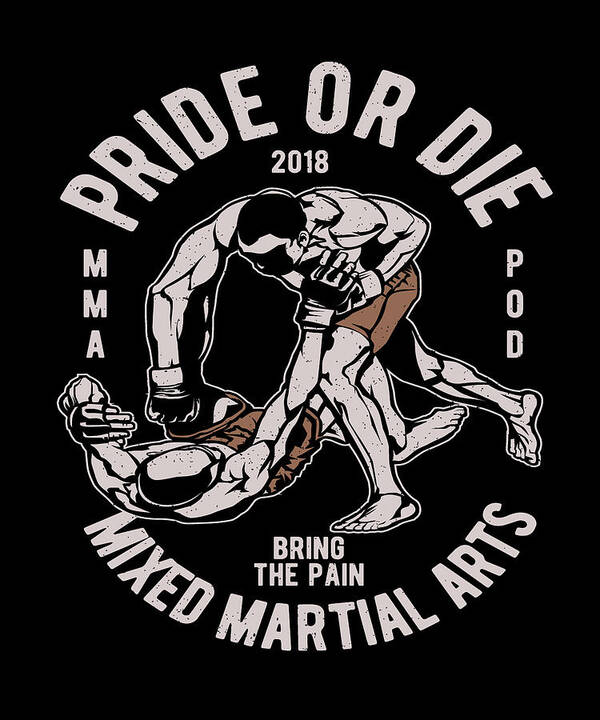This detailed poster features a striking design with a solid black background. Prominently displayed at the top in all caps and white letters, adorned with subtle black speckles, is the text "PRIDE OR DIE" curved across the center. Beneath this, "2018" is clearly printed. On the left side, the acronym "MMA" is vertically aligned, while on the right side, "POD" is similarly positioned.

Taking center stage in this image is an animated depiction of a Mixed Martial Arts (MMA) fight. Two muscular fighters, both shirtless and wearing brown (or orange) shorts, are engaged in intense combat. The fighter on top is delivering a punch to the one lying on the ground. Notably, the top fighter is wearing boxing gloves, although the gloves are absent on the downed fighter attempting to defend himself.

At the bottom of the poster, the text "MIXED MARTIAL ARTS" is elegantly curved upward, with "BRING THE PAIN" above it in slightly smaller font. This illustration, while not hyper-realistic, effectively conveys the raw intensity of the sport. The overall layout, including the vertical text and the central action, gives the poster a dynamic and engaging appearance, suitable for a banner, poster, or even apparel.